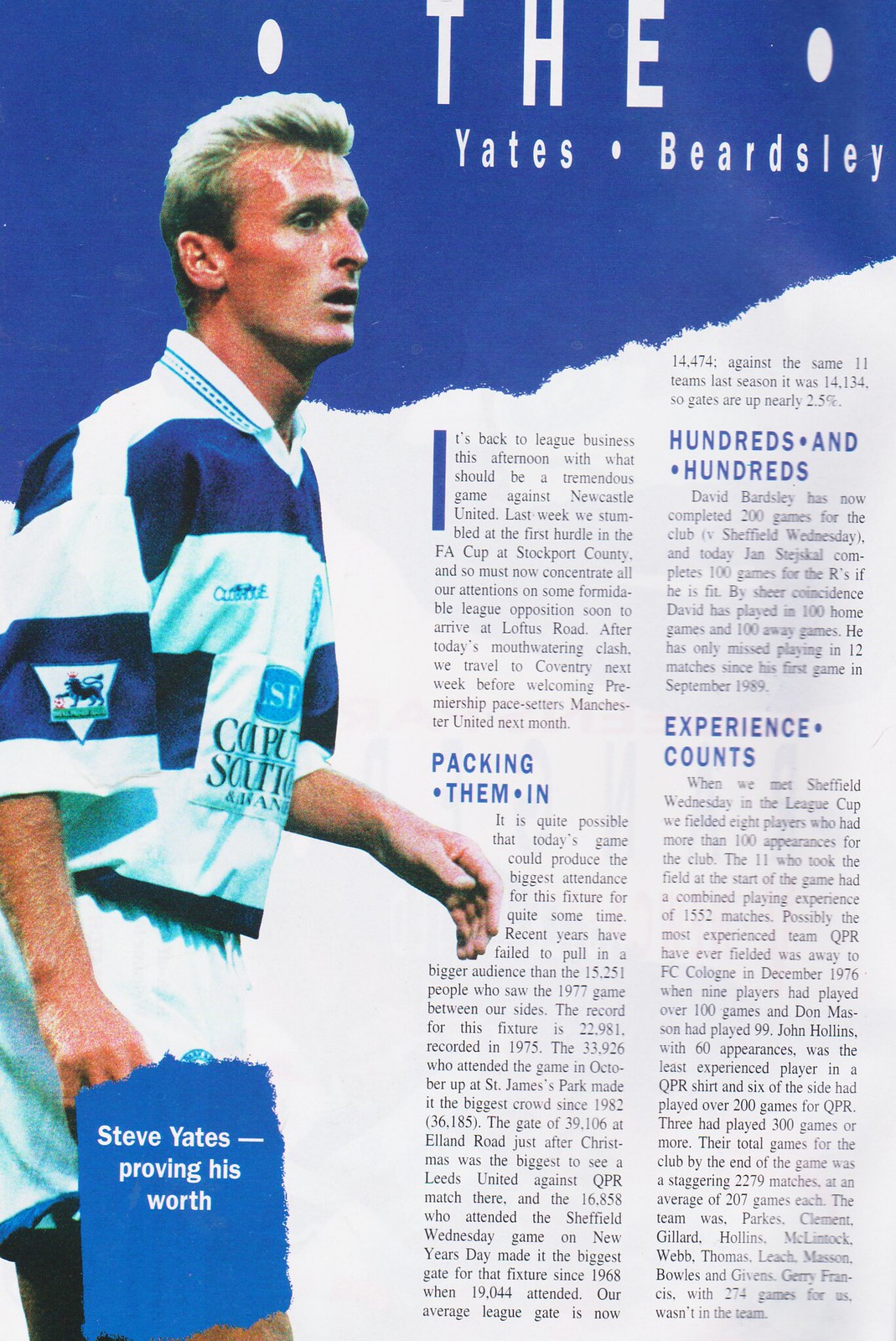This magazine page features an article centered on a soccer player, Steve Yates. The page, which appears to be from the inside of a sports program or magazine, is designed with a blue top section that transitions into a white background via a torn border effect. At the top of the page, in white text against the blue background, it reads "The Yates • Beardsley," adorned with small white dots flanking the words. The main visual element is a striking image of Steve Yates on the left-hand side. He is a white man with a flushed red face and combed-back blonde hair that darkens towards the back. Yates is dressed in a white and blue jersey with sleeves extending just below the elbows, likely bearing a sponsor logo.

Below his image, a bold graphic states, "Steve Yates — Proving His Worth." The right-hand side of the page is filled with dense magazine-style text broken into multiple sections. The first paragraph introduces the article, and is followed by three notable subsections highlighted in larger fonts: "Packing Them In," "Hundreds and Hundreds," and "Experience Counts."